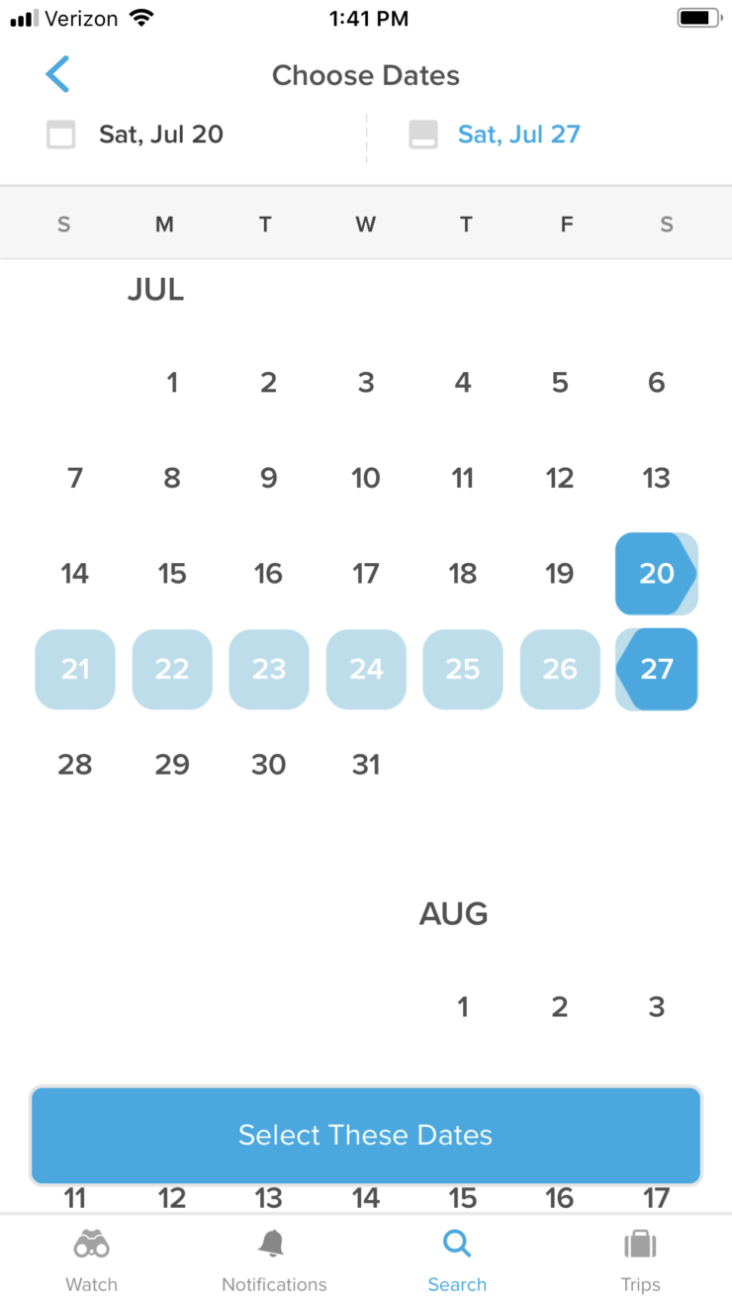This image appears to be a screenshot taken from a cell phone displaying a calendar app interface. At the top of the screenshot, there are three out of four bars of cellular service shown, labeled "Verizon," along with full Wi-Fi connectivity. The timestamp indicates that the screenshot was taken at 1:41 PM, and the battery icon suggests a charge level of roughly 75% or more, as the battery outline is nearly full. 

Centered at the top of the calendar app, "Choose Dates" is prominently displayed, accompanied by a blue back arrow on the left and a small gray calendar icon. The selected range of dates spans from "Saturday, July 20th" to "Saturday, July 27th," separated by a vertical divider consisting of five dots.

Beneath this header, the monthly calendar view is shown, starting with Sunday and ending with Saturday. The month of July is labeled, with the first day appearing on a Monday and the month concluding on the 31st, followed by an introductory view of August.

At the bottom of the interface, "Select These Dates" is displayed as a call to action. Additional navigation icons include a binoculars icon for "Watch," a bell icon for "Notifications," a magnifying glass for "Search" highlighted in blue, and a suitcase icon labeled "Trips."

This detailed caption provides a comprehensive overview of the key elements and layout of the calendar app screenshot.